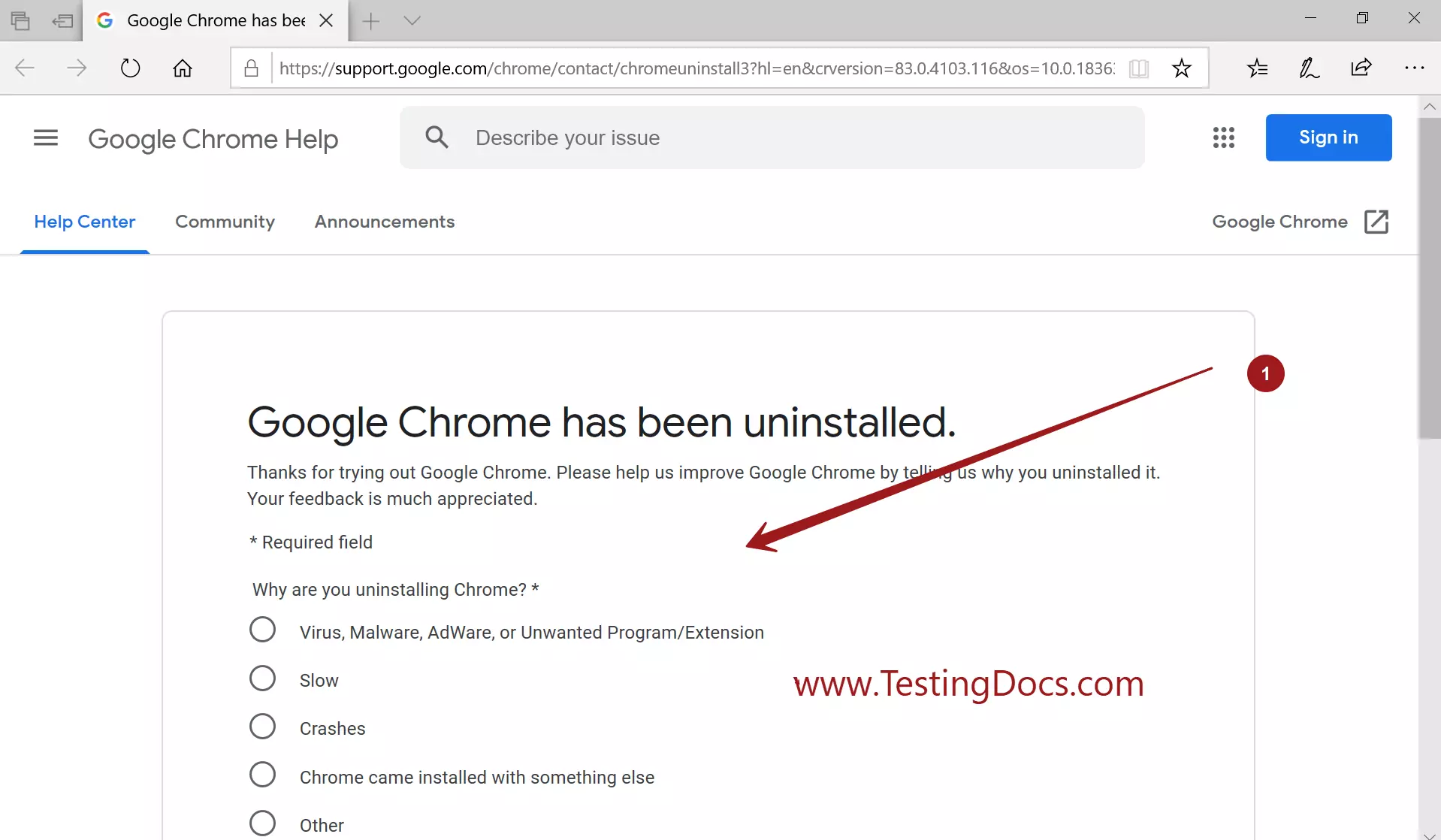This is a detailed screenshot from the Google Support website specifically focused on Google Chrome Help. The browser tab on the top left corner partially displays the title "Google Chrome has bit," with the rest of the text cut off. The URL present in the address bar reads, "https://support.google.com/chrome/contact."

The main content area is titled "Google Chrome Help." Located to the right of this title is a search box with the placeholder text, "Describe your issue." Adjacent to the search box, there is an icon consisting of nine small squares arranged in a three-by-three grid, likely indicating additional Google Apps or services. To the far right of this array is a blue "Sign In" button.

On the left-hand side of the page under the title, there are three clickable options: "Help Center," "Community," and "Announcements." Dominating the central part of the page, the text reads as follows: "Google Chrome has been uninstalled. Thank you for trying out Google Chrome. Please help us improve Google Chrome by telling us why you uninstalled it. Your feedback is much appreciated. * Required field"

Following this message is a prompt, "Why are you uninstalling Chrome? *" with five multiple-choice options for the user to select from:

1. Virus, Malware, Adware, or Unwanted Program/Extension
2. Slow
3. Crashes
4. Chrome came installed with something else
5. Other